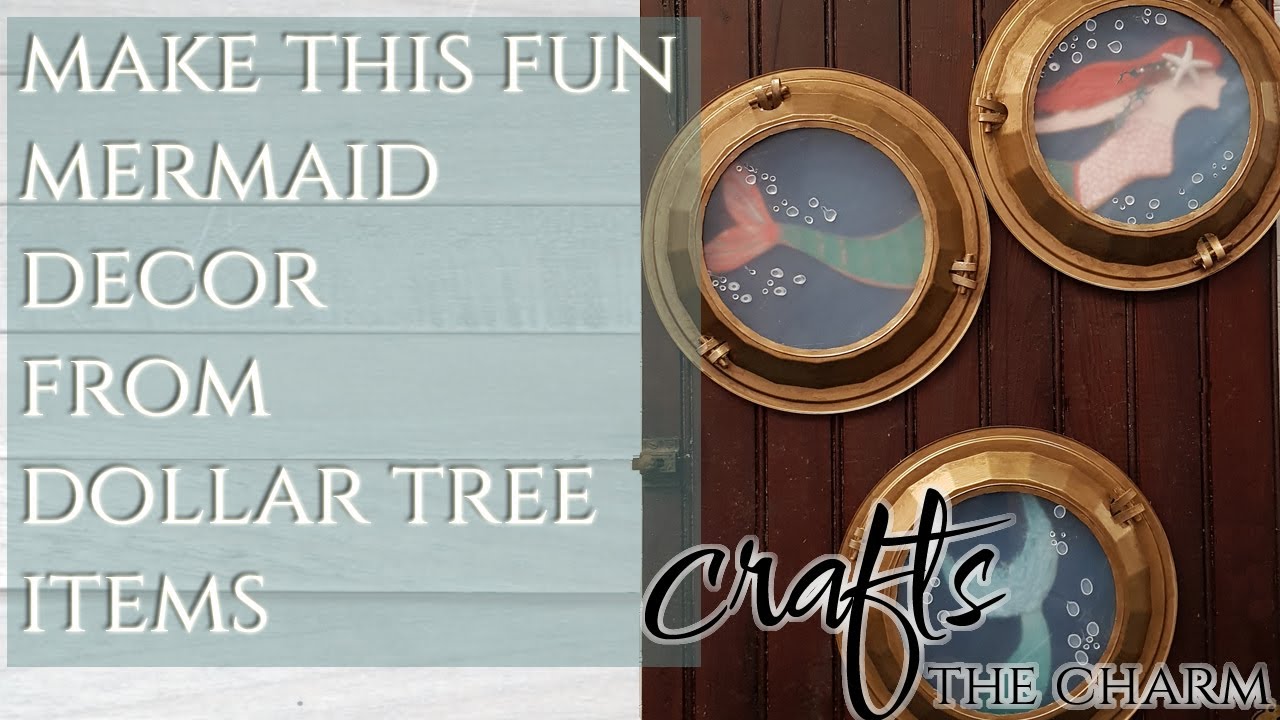This image is an advertisement for Dollar Tree, showcasing a creative DIY project for mermaid decor. The left side of the picture features a translucent gray box with white all-caps text that reads "Make This Fun Mermaid Decor from Dollar Tree Items." On the right, set against a dark brown wall with vertical wooden slats, there are three brass-colored portholes, resembling those on a ship or submarine. Each porthole features a different segment of a mermaid with flowing red hair, a starfish in her hair, and a green tail. The top porthole shows her head and upper body, the middle one displays her midsection with the continuation of her tail, and the bottom porthole focuses on the tips of her tail fins amidst bubbles. The text "crafts" appears in a script font, and "the charm" is written in all caps at the bottom right of the image.